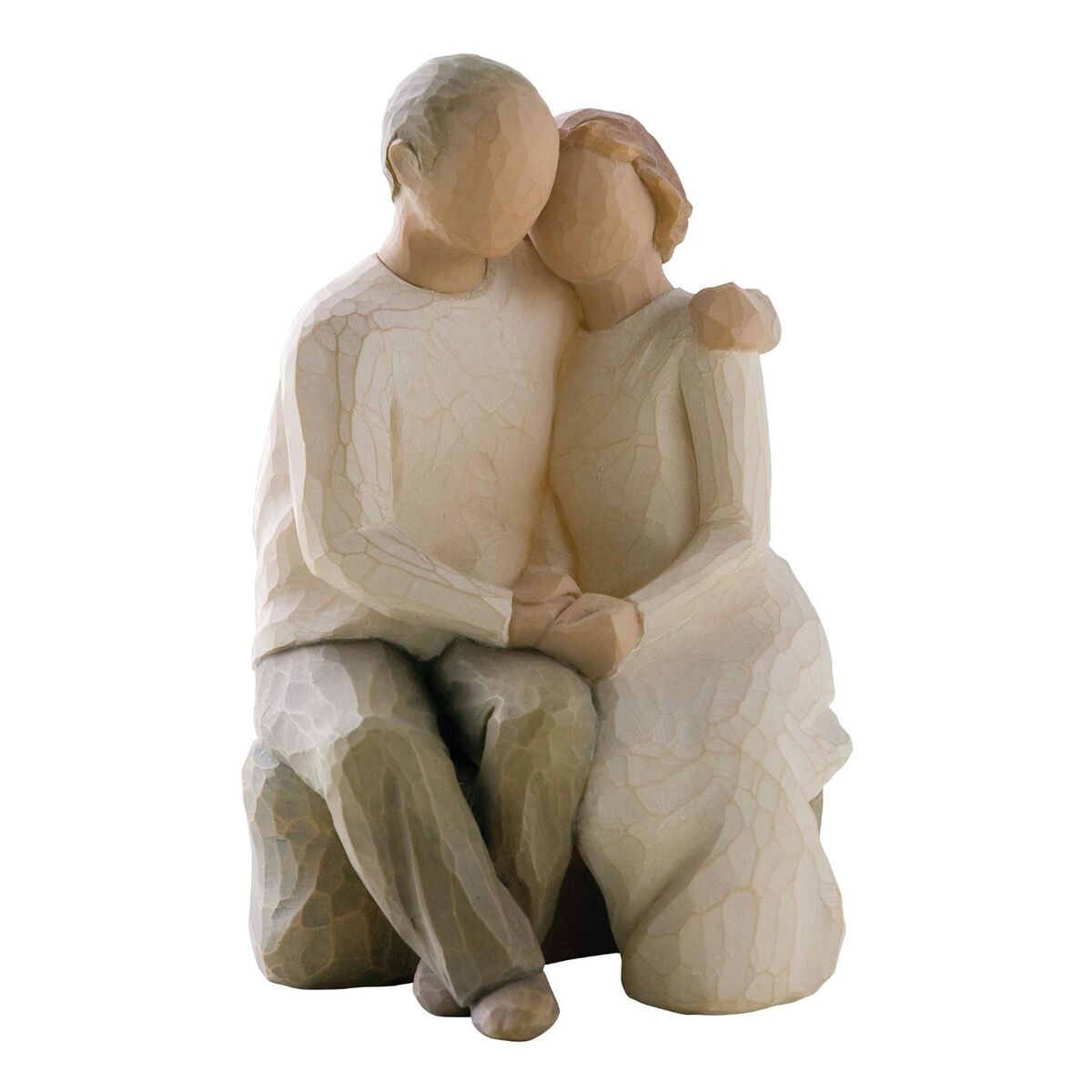This image features a detailed and angular sculpture resembling a wood carving, displayed against a white background. The artifact departs from traditional realism, with the faces of the figures lacking defined features. The sculpture depicts a man and a woman seated together on a rock or log, embracing tenderly. The man, positioned on the left, is characterized by his short, receding gray hair and is dressed in a cream-colored long-sleeve shirt, gray pants, and brown shoes. He cradles the woman with his left arm around her shoulder, while their right hands are clasped together resting on his lap. The woman, positioned on the right, has short brown hair and wears a full-length, long-sleeve gown painted in beige or white. She leans her head affectionately on his shoulder and places her left hand over their joined hands, adding a sense of unity to the scene. The overall palette of the sculpture includes natural earthy tones, emphasizing the carved texture while imparting a subtle, painted finish.